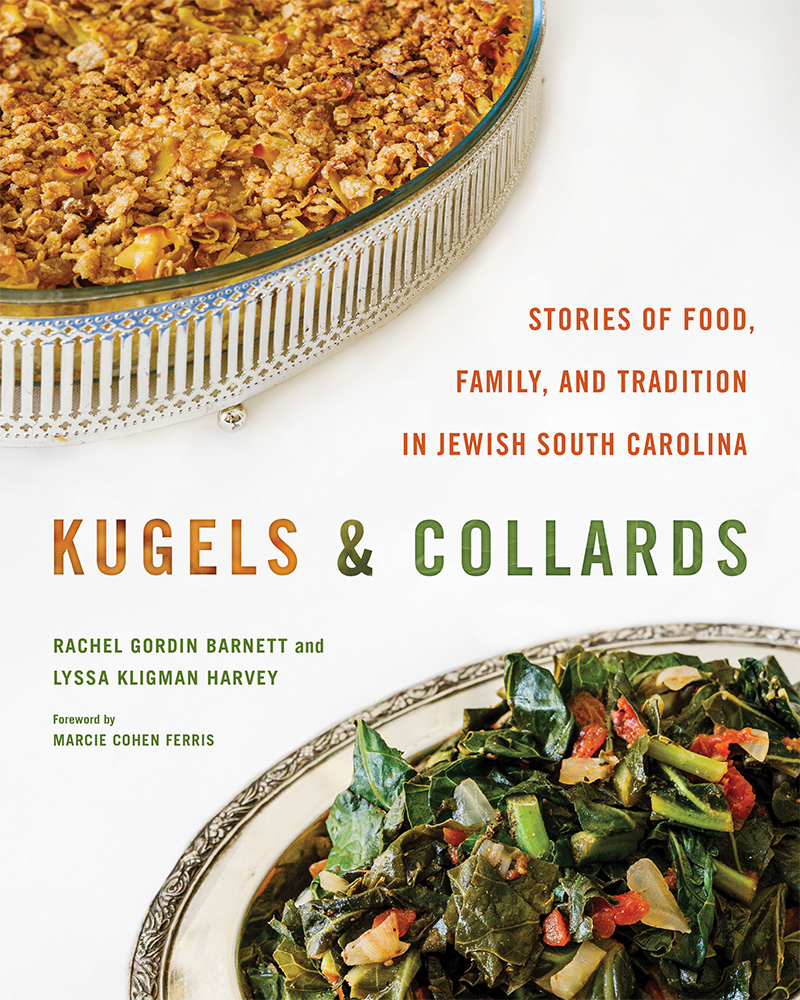The cover of the book features a vivid, colored photograph set against a white background. Dominating the top left corner is a glass dish encased in an ornate silver bowl. This dish appears to hold a brown, crispy casserole, possibly topped with nuts. Inscribed across the middle of the cover, slightly to the right, is the title in bold red and green letters: "Kugels" in red and "and Collards" in green. Above the title, in red text, it reads, "Stories of food, family, and tradition in Jewish South Carolina." Below the title, the authors' names, Rachel Gordon Barnett and Lisa Kligman Harvey, are presented in green text, followed by a foreword by Marcy Cohen Ferris. In the bottom right corner, a decorative plate with an intricate leafy border displays a vibrant salad containing dark leafy greens, possibly collard greens or spinach, mixed with pieces of red pepper and other vegetables.